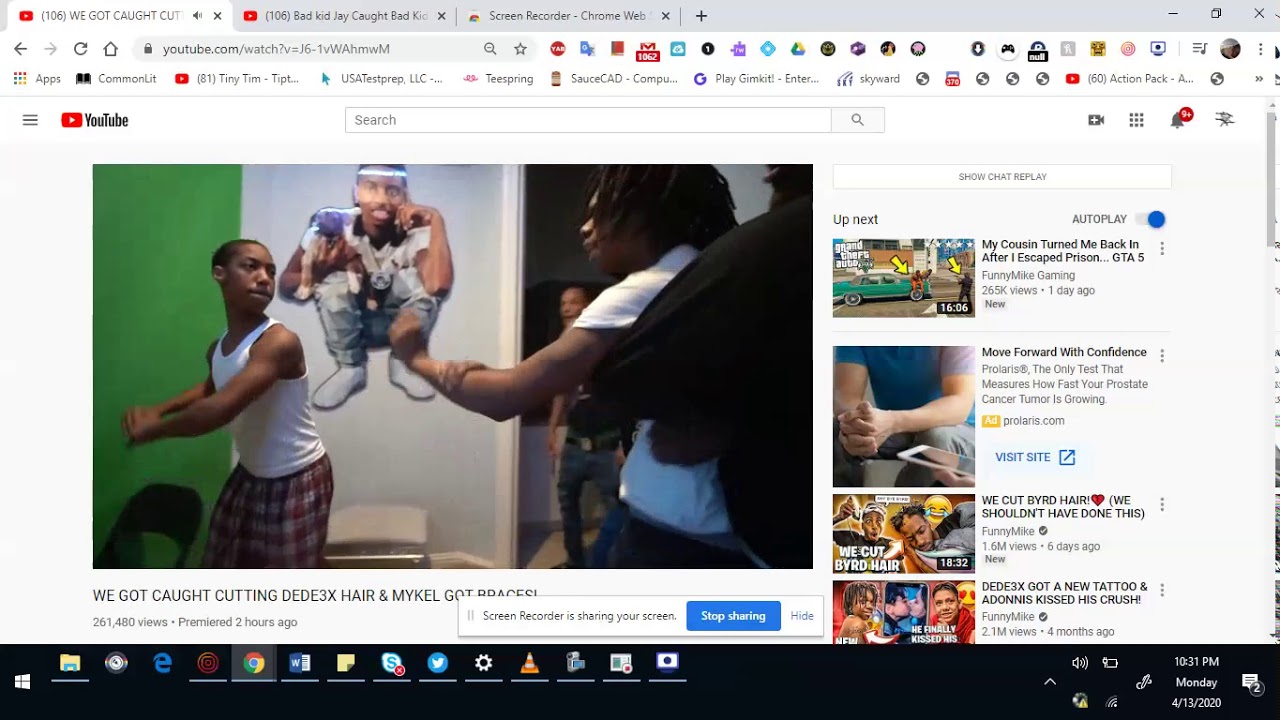Here's a cleaned-up and detailed caption based on the provided description:

---
This YouTube webpage showcases a video as its main content, displaying two Black men engaged in a fight. The foreground features a younger teenager attempting to intervene, whilst an adult man is restrained by another individual. In the background, another onlooker is present. Edited into the scene is an image of a Black man squatting with his cheek resting on his hand, looking amused. The video is titled "WE GOT CAUGHT CUTTING DEDE3X'S HAIR, AND MICHAEL GOT BRACES," in bold black text. On the right side of the screen, a vertical list of upcoming videos from an autoplay playlist is visible. A black ribbon stretches across the bottom of the screen, displaying the time "10:31 p.m." and the date "Monday, April 13, 2020." Various icons such as File Explorer, Internet Explorer, Chrome, Word, Skype, and Twitter settings are aligned to the left of the ribbon.

---

This rewritten caption maintains the organization and detail for clarity and readability.